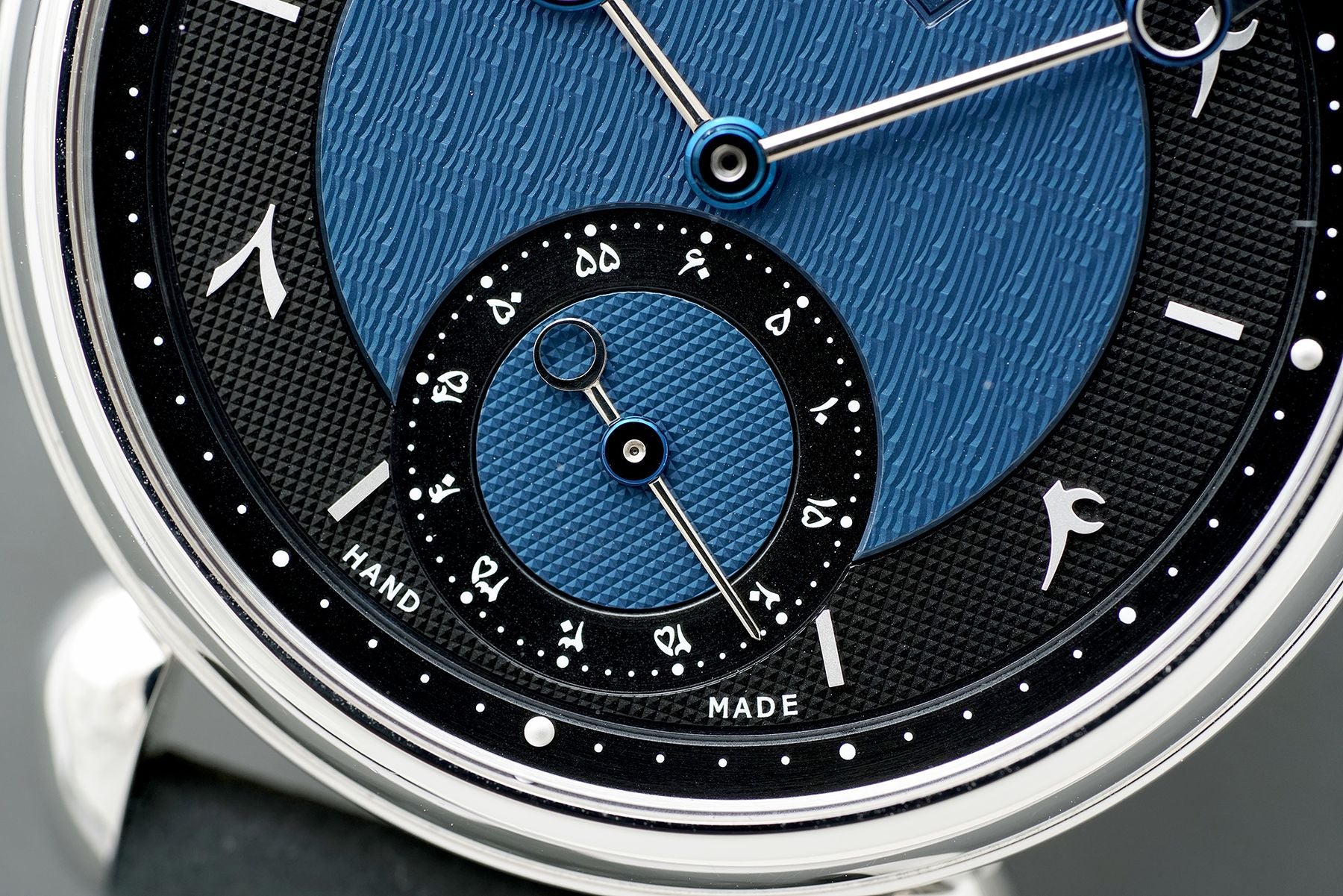This detailed photograph showcases the face of a luxurious, handmade watch. The zoomed-in image depicts the watch face with meticulous clarity, highlighting the unique design and craftsmanship. The watch features a steel outer frame with a black lining marked with degree dots, presumably for rotational reference. The main dial of the watch has a striking blue center surrounded by a black backdrop. 

Intriguingly, the watch lacks conventional numbers or Roman numerals; instead, each hour is marked by distinct symbols. For instance, the three o'clock position is indicated by a horizontal slash, while the four o'clock position resembles a metal bottle opener. The large hour and minute hands are crafted from silver, and there is an additional smaller dial within the main face, possibly indicating seconds, although the exact purpose is unclear.

All the text and symbols, except for the word "handmade," are in a foreign language, adding an exotic touch to the watch's design. The only legible line in English, "handmade," is prominently displayed at the bottom of the watch face, emphasizing the artisanal quality of this exquisite timepiece.